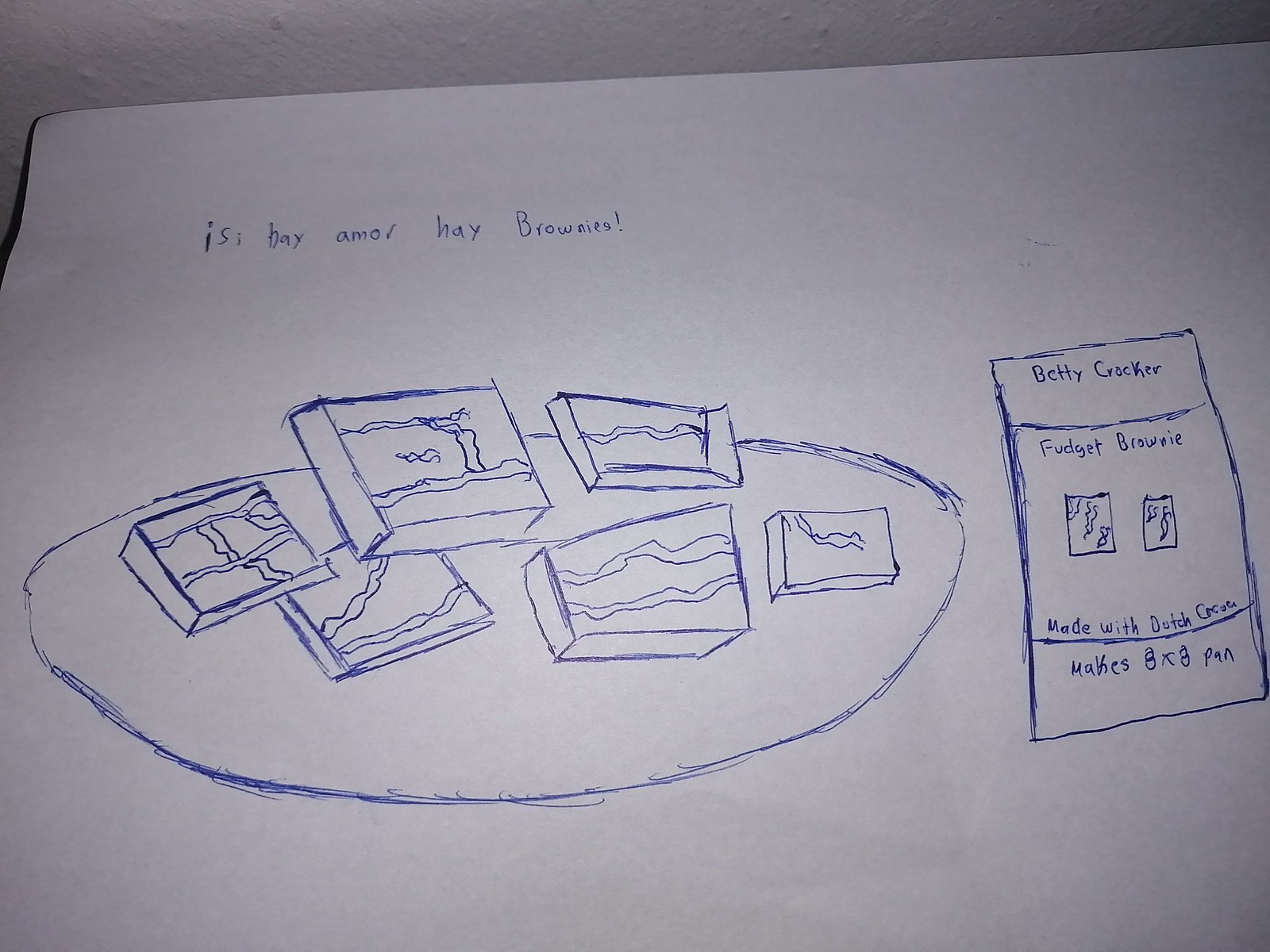This detailed illustration, executed with blue ink, depicts a plate adorned with small boxes, each containing intricate squiggly patterns. Above the plate, a Spanish phrase is inscribed, which appears to be "Sí, amo estos brownies" (Yes, I love these brownies). To the right of the plate, there is a depiction of a brownie package, resembling Betty Crocker Fudge Brownie mix. The package features similar squiggle designs and inscriptions highlighting "Made with Dutch Cream" and "Makes 8x8 Pan". The entire illustration is set against a white sheet of paper, with a white wall serving as the backdrop.